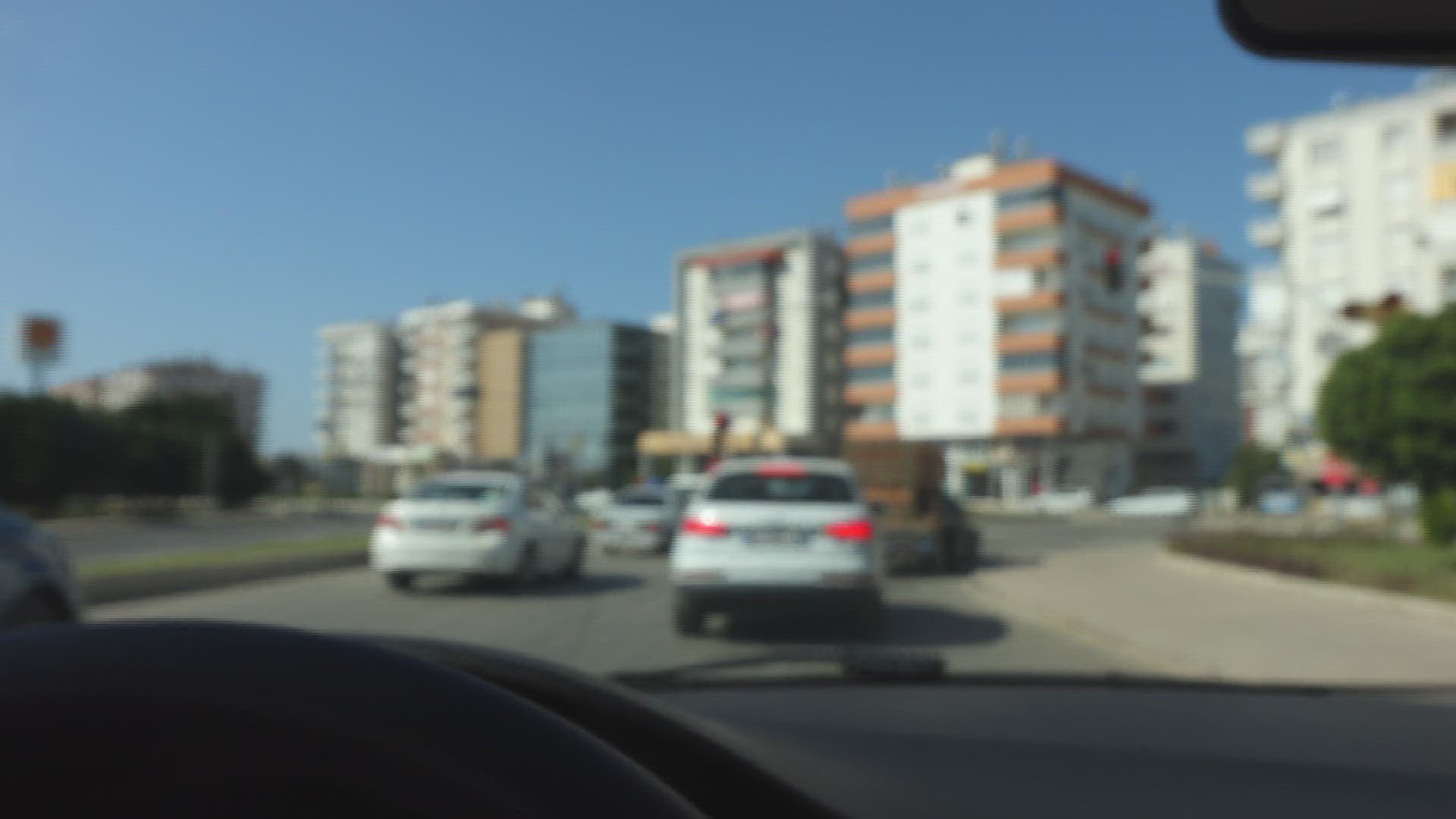In the foreground, three white cars are lined up, with one of them prominently displaying red taillights. Positioned in front of this car is a sizable brown box, underneath which a smaller brown car is partially visible. The backdrop features a series of buildings: a white building, a brown-and-white building with distinct horizontal brown levels and a white center section, another white-and-brown building, a blue building, a tan building, and several additional white buildings. Surrounding the scene on both sides are lush green trees. The sky above is a clear blue, providing a striking contrast to the gray pavement and sidewalks below. The grass is a vibrant green, adding to the overall vividness of the scene.